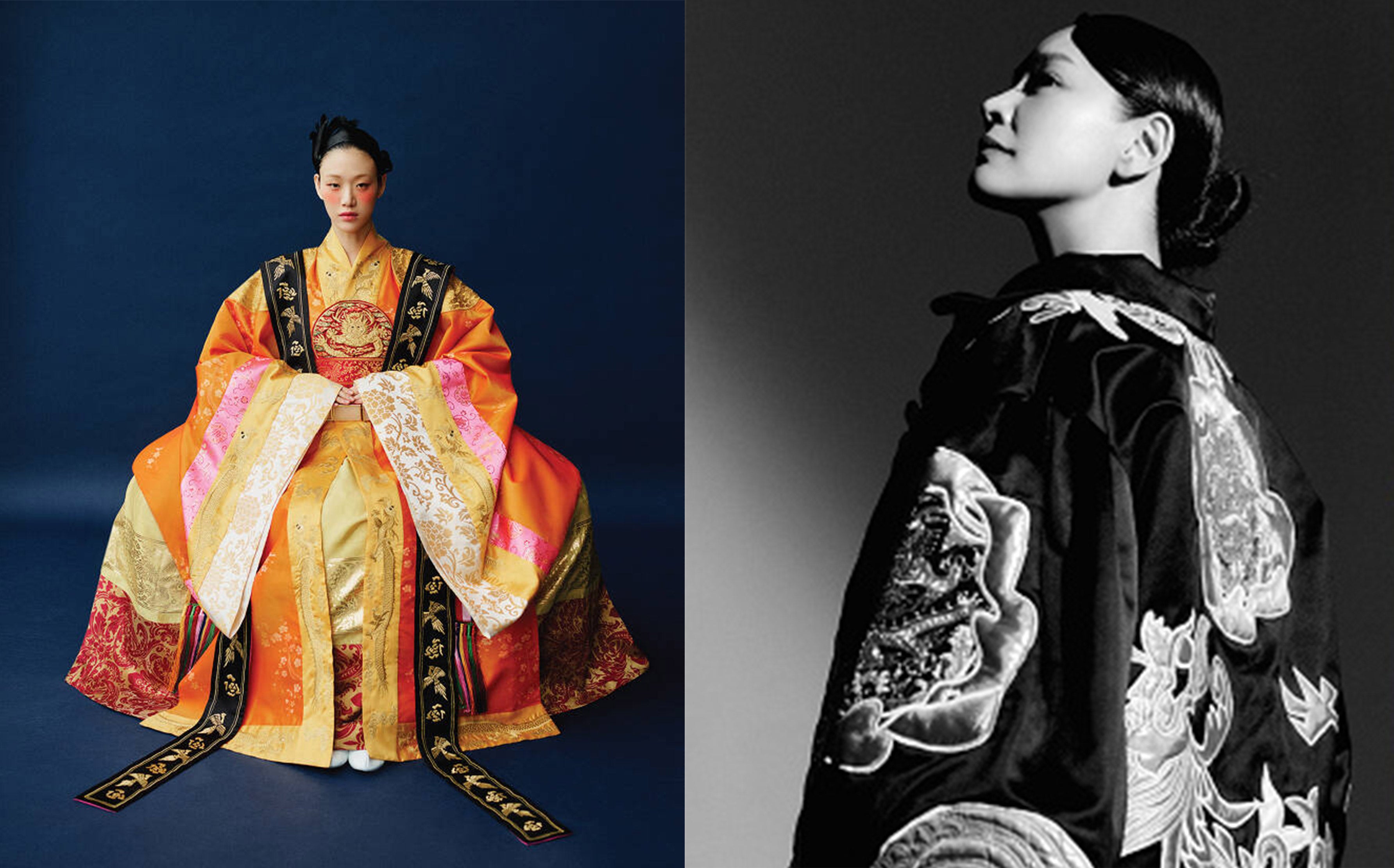The image features two photographs of a Japanese woman, each depicting different styles and contexts. The left photograph is vibrant and colorful, showcasing the woman seated on a blue floor with a matching blue background. She is adorned in traditional Japanese attire, commonly known as a kimono, which is exceptionally large and ornate, enveloping her entirely. The kimono displays a rich palette of orange, red, gold, pink, ivory, and tan, with intricate floral and embroidery patterns. A striking black and gold inlaid sash, bearing Japanese writing, drapes elegantly around her shoulders and cascades onto the floor.

The right photograph, in black and white, offers a more subdued but still elegant depiction of the same woman. She is shown standing and looking upwards, her profile conveying a sense of grace and reflection. In this image, her robe is predominantly black with light-colored or silver embroidery, providing a sharp contrast to the vibrancy of the colored photo. The overall emphasis in the black and white image shifts to the woman's expression and posture, highlighting her serene presence.